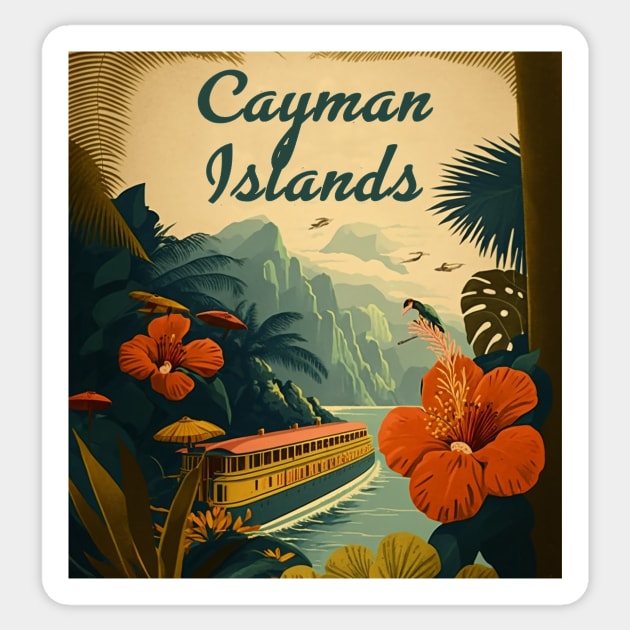This image, reminiscent of vintage 1940s advertising art, displays an illustrated promotion for the Cayman Islands. At the top, "Cayman Islands" is elegantly scripted in green, set against a muted yellow sky. The scene features a river flowing through the center, where a ferry boat sails peacefully. Surrounding this central waterway are lush jungle elements—vibrant red flowers, dense fern leaves, and towering palm leaves. Green mountains flank the sides of the river, while a cloud-covered mountain peak rises in the background. The illustration is framed by a white border, enhancing its presentation as a card or perhaps a vintage-style coaster, with sepia tones giving it an antiquated feel. Birds soar above the tranquil scene, adding to the idyllic depiction of this tropical paradise.